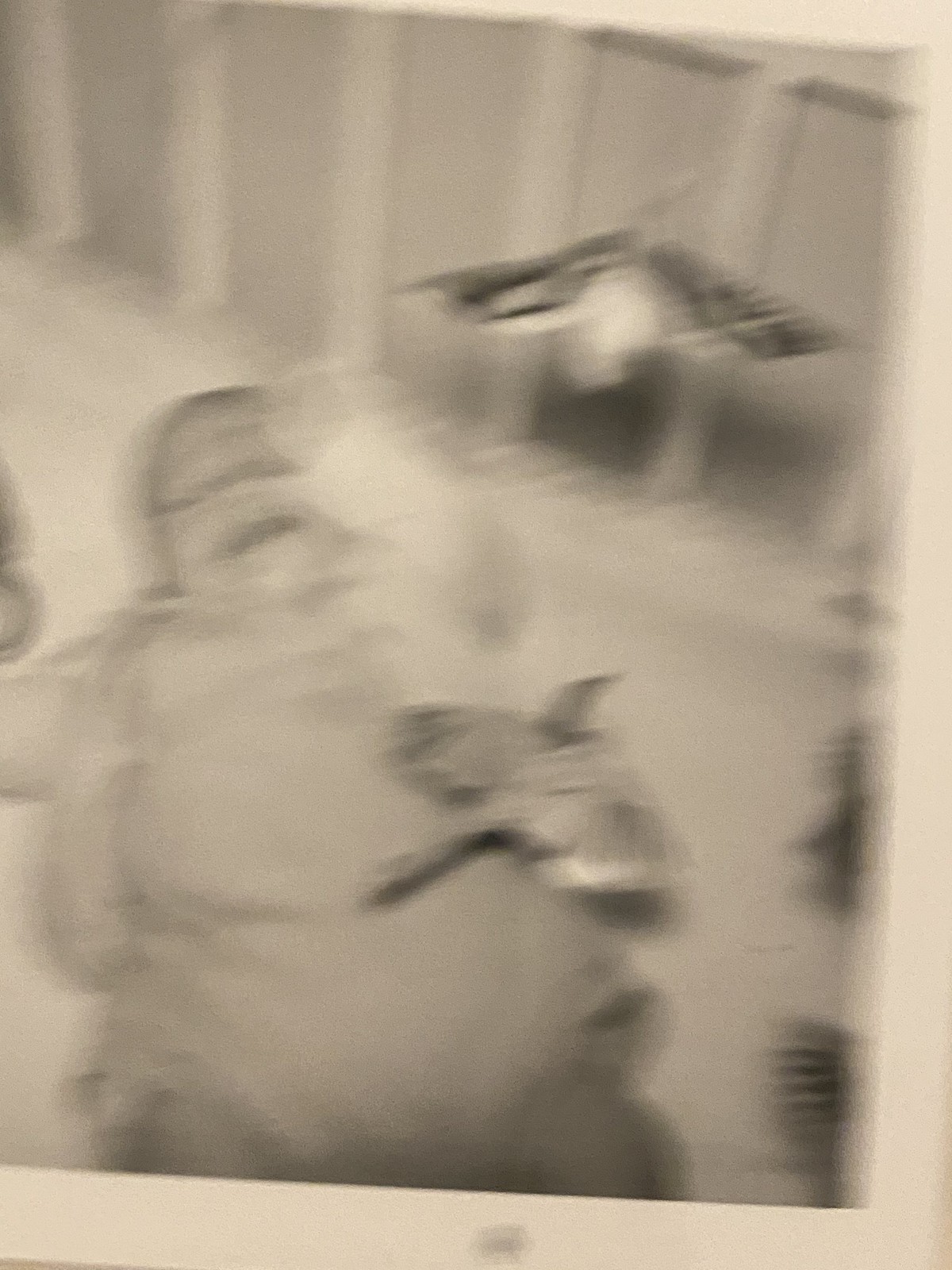This photograph, printed on tan or beige paper, evokes an antique or retro style. It is an extremely blurry and distorted black-and-white image, capturing a baby lying on its back in a crib. The crib, which has white bars, holds the baby dressed in a light-colored onesie with short legs. The baby appears to be in distress with its mouth open as if crying and has its left hand raised near its face. A thin covering of hair is visible on the baby's head. The crib’s sheet or blanket also appears to be white. In the crib, there appear to be two bird-like shapes, possibly part of a mobile, with one positioned above the baby's head and another near its right hip. These objects may be toys but resemble real birds under the poor image quality. Reflective areas are also noticeable in the photograph, which is taller than it is wide.